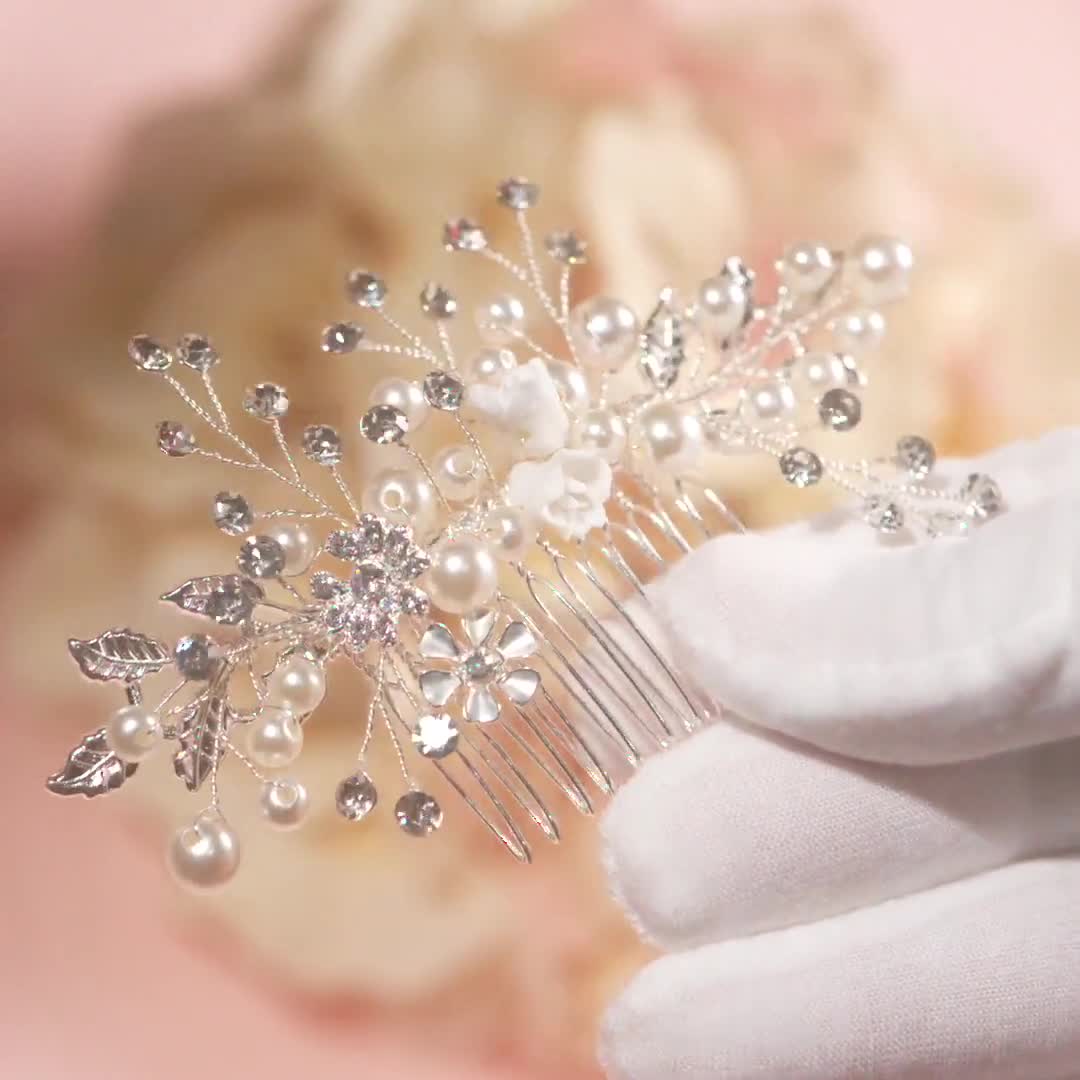The photograph captures a highly detailed, close-up image of an ornate hair clip held by gloved fingers positioned in the bottom right corner of the frame. The gloves are white fabric, ensuring a clear view of the exquisite hair clip centered in the image. The hair clip boasts an intricate design featuring a silver metallic base adorned with black leaf patterns, silver flowers, cream-colored pearls, and crystal-like studs. These decorative elements are artistically arranged to resemble branching twigs with budding pearls and mini petal flowers. The bright lighting accentuates the clip's luminous and reflective qualities, enhancing the clarity of the image. The blurred background exhibits shades of pink and light brown, adding a soft contrast that keeps the focus on the intricately designed hair clip.